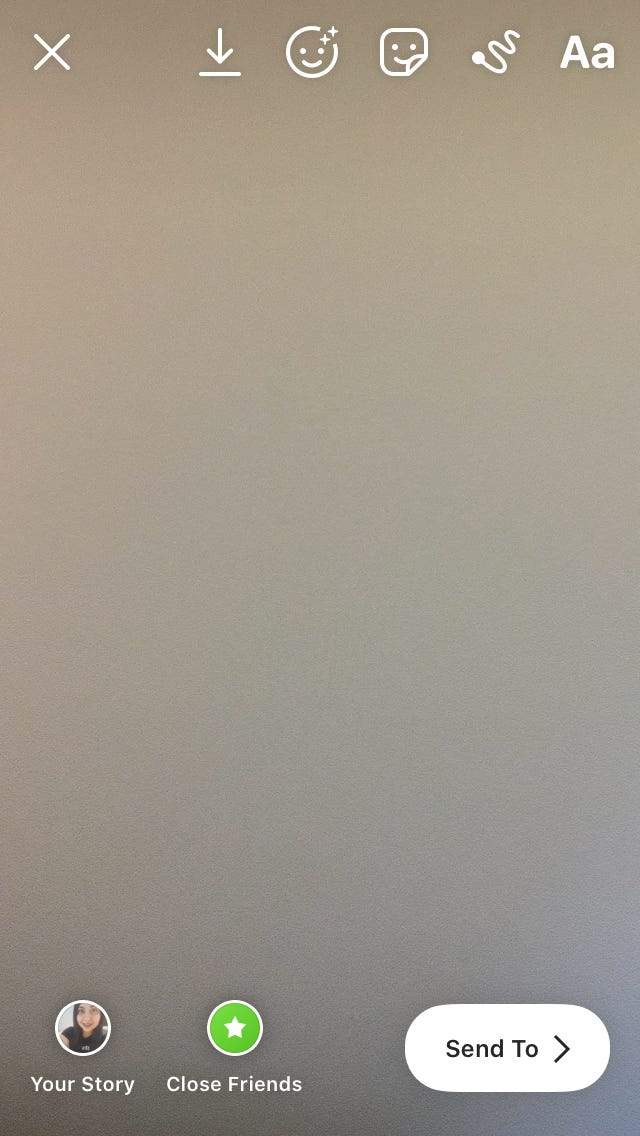A screenshot resembling a common social media interface is displayed. In the upper left-hand corner, there's a prominent white "X" icon. Adjacent to this, a download button can be seen. On the interface, there is a circle icon featuring a smiley face adorned with sparkly accents, alongside a sticker also depicting a smiley face. A squiggly line icon, often used for drawing, is present next to an icon representing text, marked by the letter "A".

The central portion of the interface showcases a beige background that transitions into a blue gradient towards the bottom right corner. In the bottom left, there is a circular avatar icon labeled “Your Story” which shows an individual with pale skin, brown hair, and a black shirt. Beside this, another circular icon labeled “Close Friends” is set against a green background with a white star in the center. To the far right, a button labeled “Send To” features black text on a white background with a rightward pointing arrow.